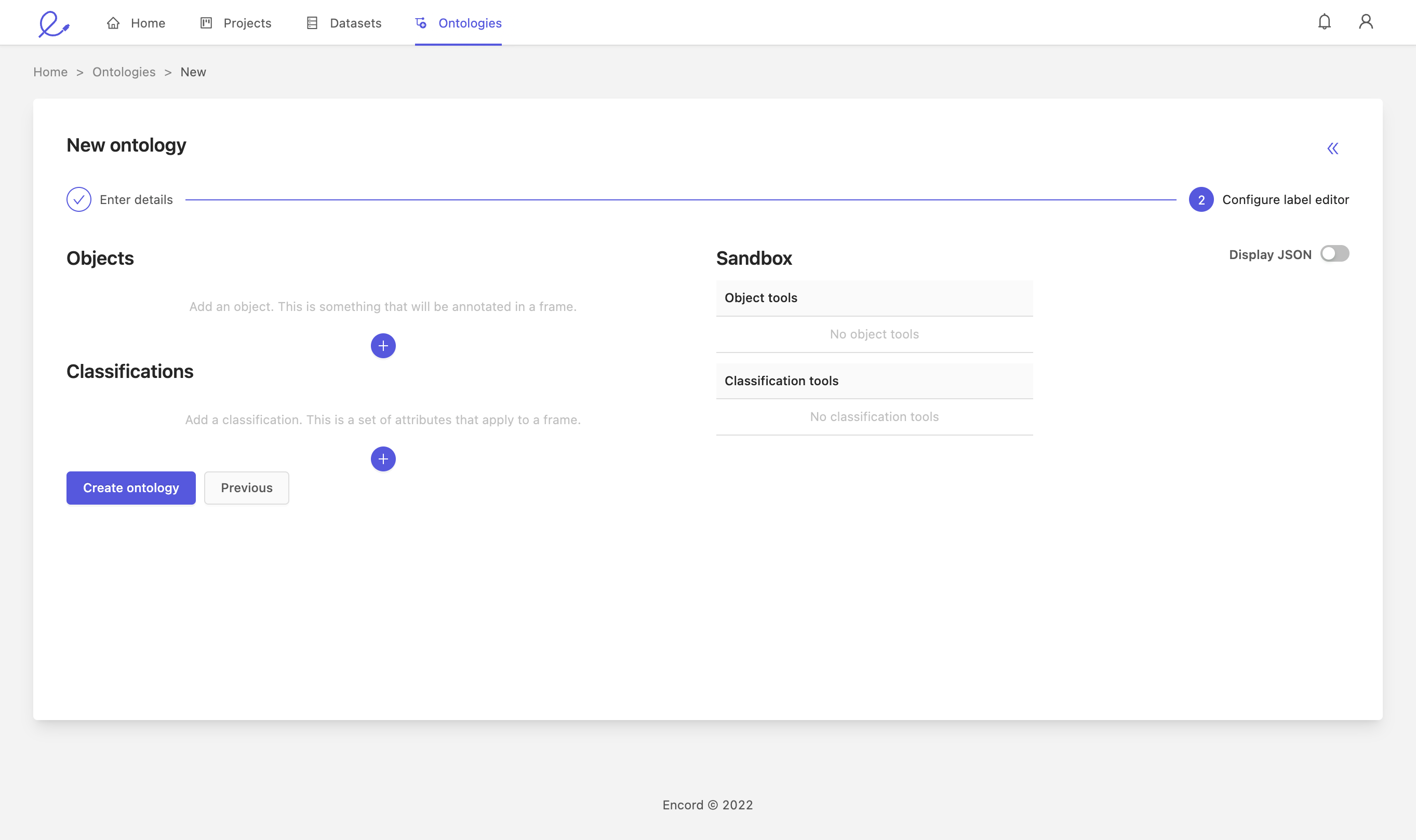Screenshot from a Customizable Process-Related Web Page

This screenshot captures a webpage that appears to be associated with process customization or testing, viewed in landscape orientation without defined borders. The webpage seems to be accessed via a desktop or laptop computer.

At the very top, there is a white border featuring a squiggly line resembling the letter 'E,' rendered in a purplish-blue font. Adjacent to this are black links accompanied by icons, labeled as "Home," "Projects," "Datasets," and another link starting with an "O," which is underlined in purple and is not fully legible.

Beneath this navigation bar, a gray section dominates the page. This section includes header labels reading "Home," "Orthologies," and "New," with "New" highlighted in black. Within this gray section lies a large white rectangular box with a prominent black header titled "New Ontology." Directly below, a blue or purple circle, check-marked and set against a white background, identifies the step "Enter Details." This is followed by a long purple horizontal line, leading to another purple circle with a white number two, indicating the subsequent step "Configure Label Editor."

Further down, the interface displays sections labeled "Objects" and "Classifications," each featuring purple circles to add items. Below these sections, there is a long, purple, rectangular button labeled "Create Ontology." A white button with black text labeled "Previous" is positioned near the bottom. The remainder of the page appears to consist of white space interspersed with a few additional boxes.